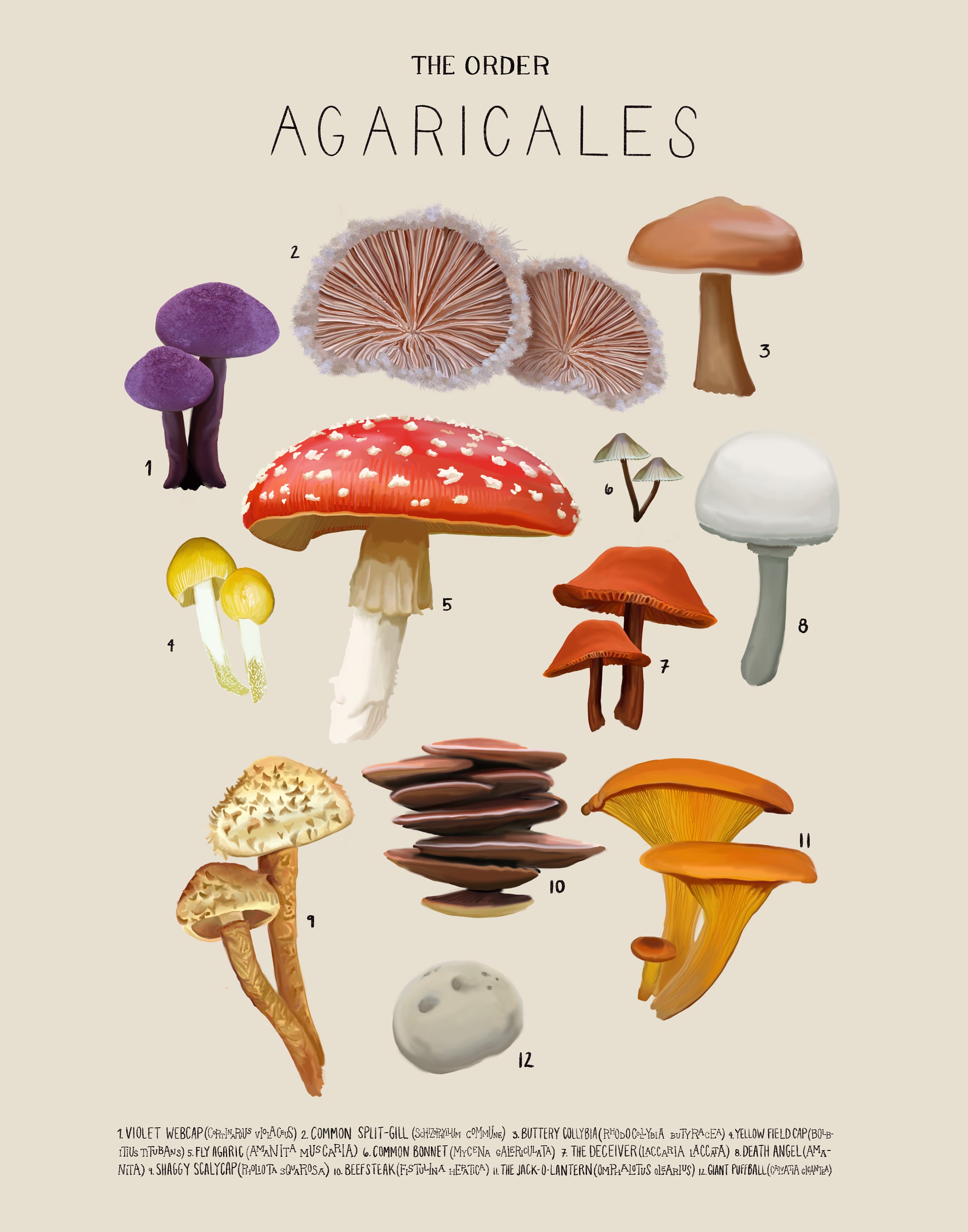This vertical rectangular poster features a light beige background and an array of twelve different mushrooms, each uniquely numbered from 1 to 12. At the top of the poster, bold black letters spell out "Agaricales," signifying the order of the fungi displayed. 

The mushrooms vary in color and shape, offering a colorful and fascinating glimpse into fungal diversity. Number 1 showcases yellow-capped mushrooms, while Number 2 features pink and white capped mushrooms with a visible underside. Number 3 is a tan-colored mushroom, and Number 4, although not described in detail, carries its own distinct appearance.

Number 5 highlights the well-known Amanita muscaria, easily recognizable by its red cap adorned with white specks. Number 6 depicts smaller mushrooms that are white and gray with black stems, and Number 7 includes another red variety. Number 8 is characterized by a white and gray cap.

The subsequent mushrooms continue the diversity: some are brown, white, or yellow, and there are additional descriptions of a complete white mushroom with a gray bottom and an orange cap with white spots. 

At the bottom of the poster is a paragraph in a different language, offering additional information that remains unreadable. Overall, this poster is a comprehensive display of the Agaricales order, capturing the varied and intricate beauty of mushrooms.